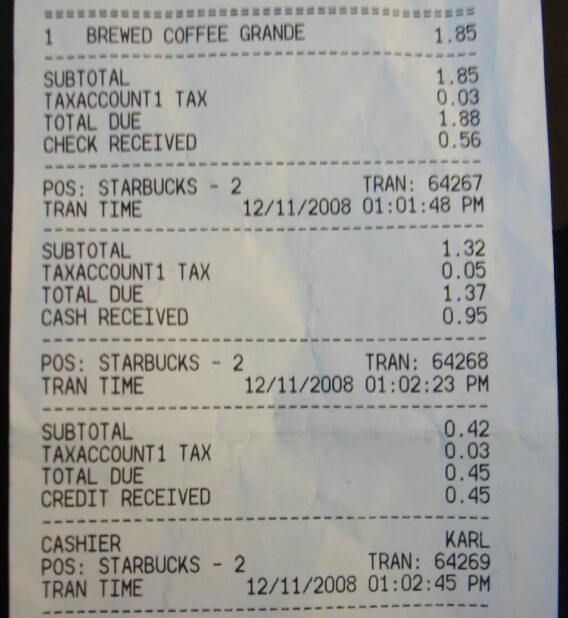The photograph depicts a detailed breakdown of Starbucks transactions printed on a white piece of paper. At the top of the page, there are light gray squares running horizontally, creating a bordered header. Directly beneath this header, there is a sequential transaction listing. The first entry starts with the number "1" in black on the left, followed by the text "BREWED COFFEE GRANDE" in all caps. Adjacent to this description, on the right edge, the price is clearly marked as "$1.85".

A dashed horizontal line separates this entry from the subtotal section below. Here, the word "Subtotal" appears on the left, with the corresponding amount "$1.85" aligned to the right. Following this, there is a line indicating "Tax Acct 1 Tax" on the left, with "0.03" (representing three cents) listed to the right.

Next, the total amount due is highlighted with the text "Total Due" on the left side, showing "$1.88" on the right. Directly beneath it, "Check Received" is printed, indicating an amount of "56 cents."

This pattern with similar entries and dashed line separators continues down the rest of the image, maintaining a uniform appearance. All the text throughout the receipt is printed in black, providing a clear and consistent depiction of the transactions.